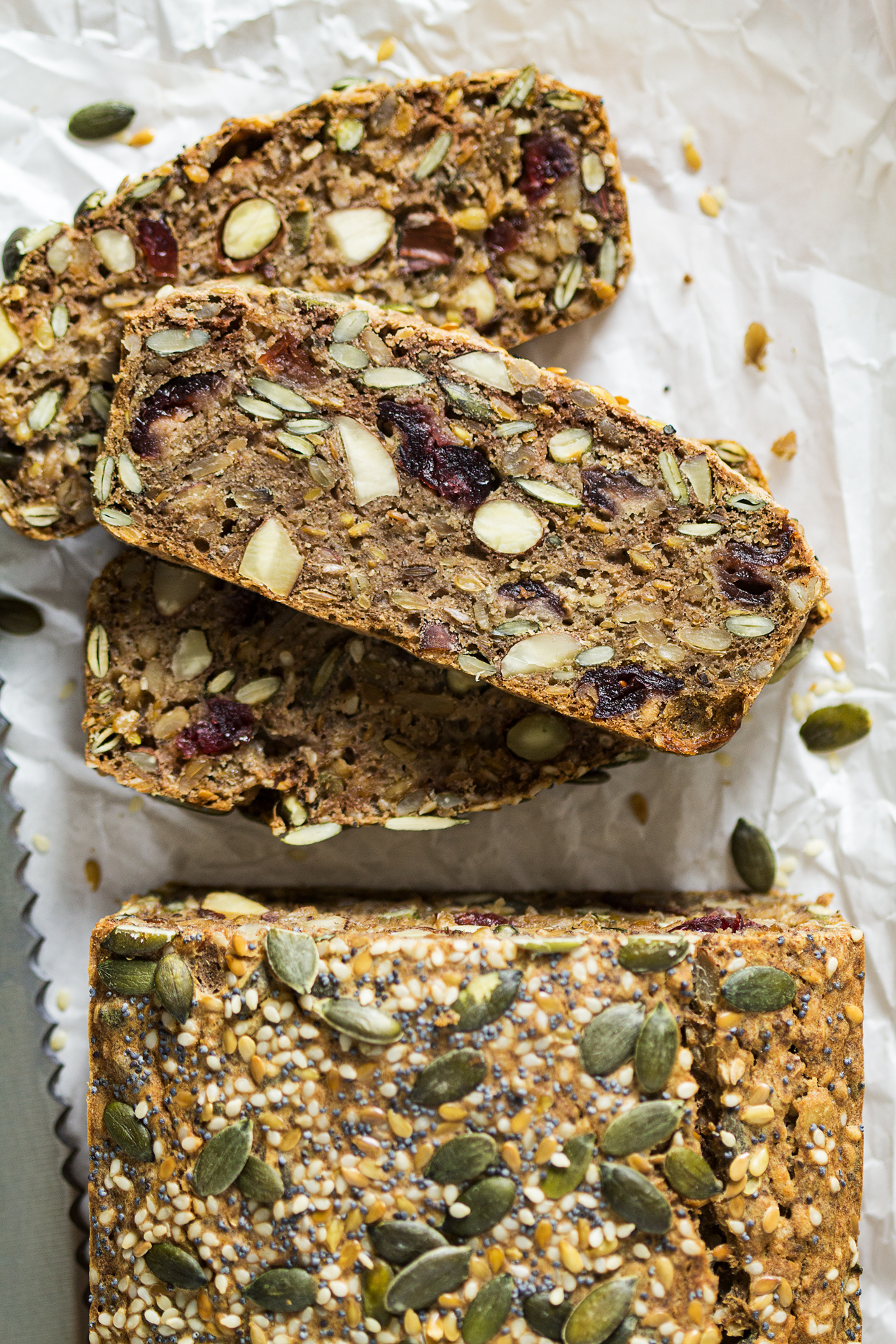This photograph captures a close-up, top-down view of what appears to be a homemade granola bar or seed bread. The dense, beige-colored loaf is richly studded with an assortment of healthy ingredients, including pumpkin seeds, sunflower seeds, sesame seeds, poppy seeds, assorted nuts, dried blueberries, and possibly dried cranberries. The bar has been sliced into three pieces, with one piece lying atop the others. The surface is adorned with a decorative interplay of seeds and nuts, creating a visually appealing mix of light brown and green hues. As crumbs and stray pumpkin seeds scatter around the bars, a gray serrated knife rests distinctly on the left side of the white wax or parchment paper, adding a touch of rustic charm to the scene.